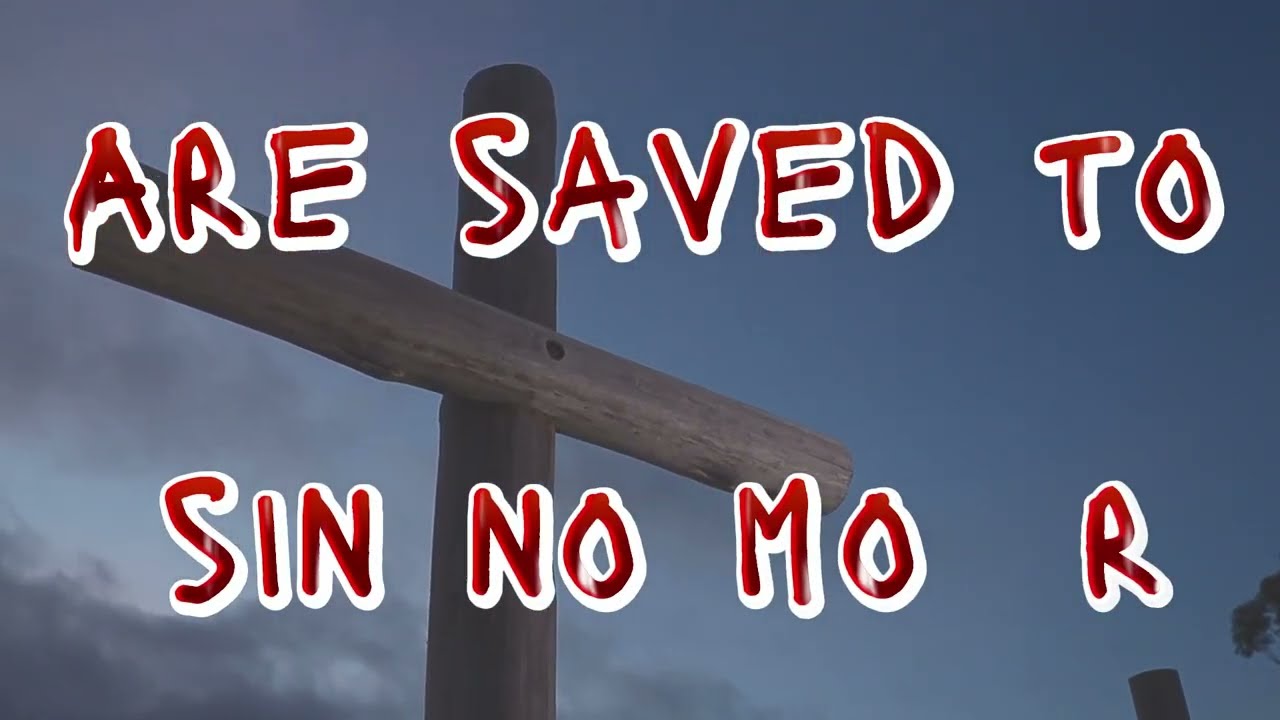This photograph showcases a wooden cross prominently featured against a deep blue evening sky, with the vantage point offering a slight upward angle as if the viewer is looking up at the cross. The cross is distinctively marked with red letters outlined in white; across the top beam, the text reads "R save 2," and below that, it spells "SIN NO MO R." The natural texture of the wood grain is visible on the cross, enhancing its rustic appearance. The sky in the background features low, hazy clouds, adding to the atmosphere of the scene. To the right side of the image, the edge of a tree is visible, and there is also what appears to be the top part of another cross, mirroring the main cross in structure.